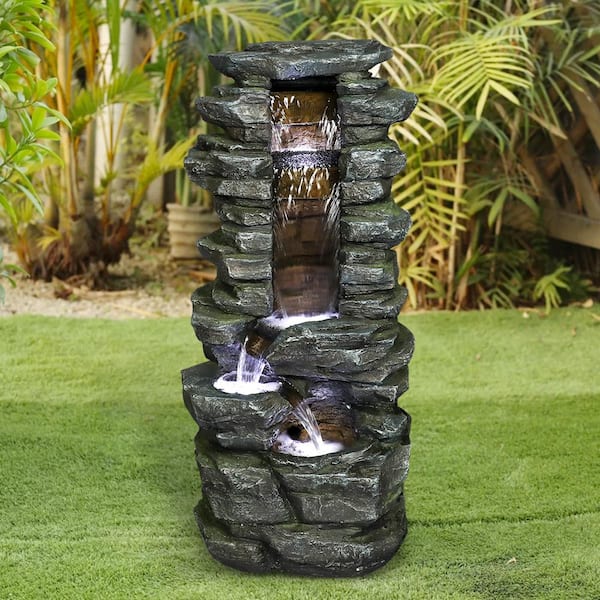In this square, daytime photo, a tall, slender fountain made of stacked, dark-colored rocks stands prominently on a well-manicured, green lawn, which appears to be artificial grass. The fountain features multiple tiers from which water cascades down in a gentle, continuous stream, creating small patches of foam as it flows. The water moves down a central channel, diverging to the left at one level and then to the right at another, before filtering back. In the background, there's a lush line of leafy Eureka palm trees, with beige stones neatly arranged at their bases, enhancing the serene backyard setting.